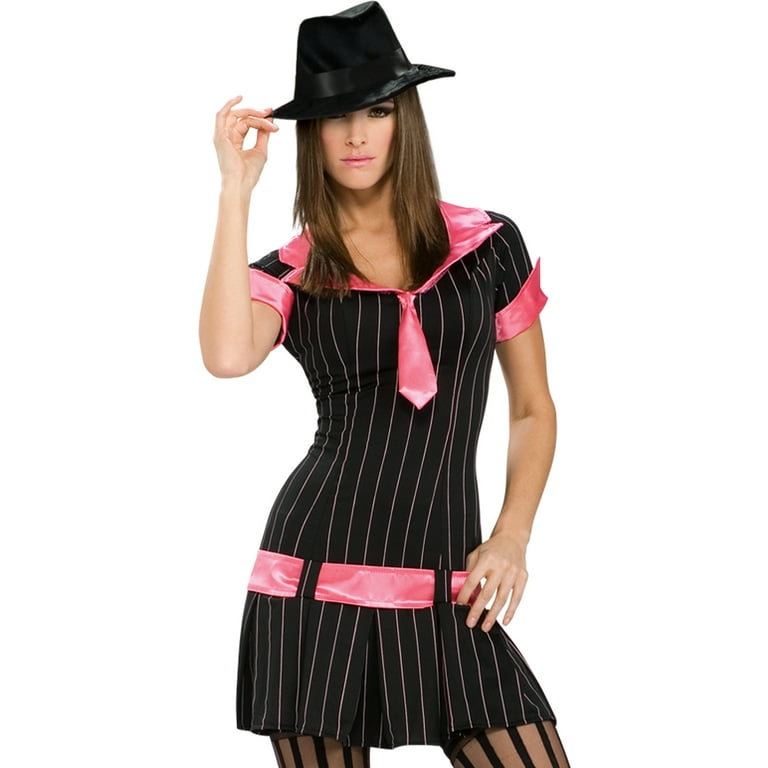The photograph features a woman wearing a tight, pinstriped black dress adorned with bright pink accents, giving her a distinct gangster-style look reminiscent of the 1950s. She sports a black, satin-like fedora, which she holds by the brim with her right hand, tipping it slightly. Her brown, medium-length hair flows down to her chest, complementing her sophisticated appearance. The dress includes a prominent pink collar that folds over, leading into a small pink tie. The short sleeves of her dress are capped with pink cuffs, matching the pink belt at her waist that loops through external belt loops, giving the dress a dropped waistline. Her left hand is resting near her belt, and she wears black striped stockings with sheer areas in between, elongating her legs. Her look is completed with pink lip gloss that matches the pink details of her outfit, suggesting a cohesive, coordinated style that might be intended as a Halloween costume, perhaps evoking a female mafia character.